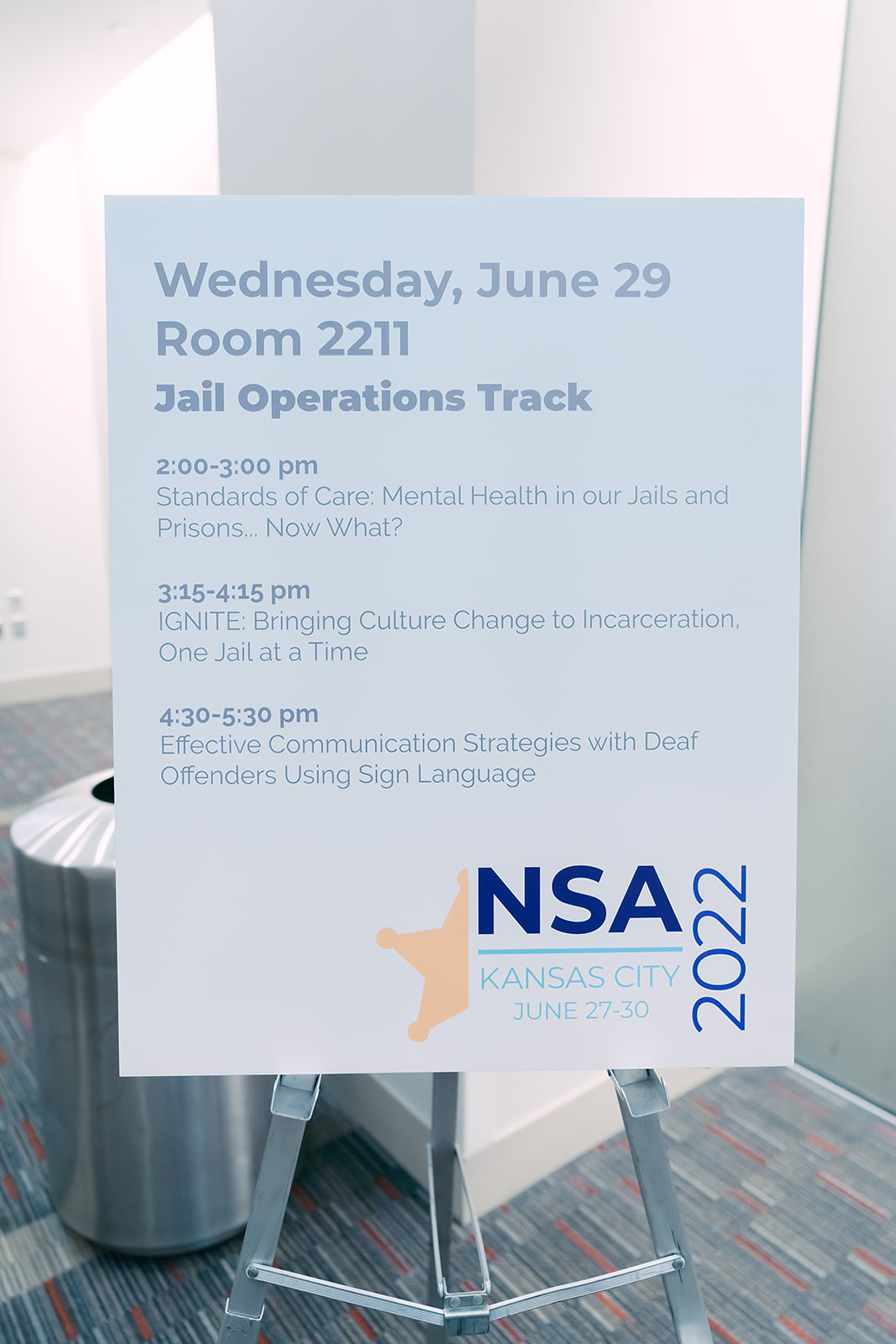The image depicts a large poster mounted on a metal tripod in a convention center or meeting area. The poster, which has a gradient design transitioning from light blue at the top to white at the bottom, details events for Wednesday, June 29th. The poster reads: 

- "Room 2211, Jail Operations Track"
- "2:00 PM - 3:00 PM: Standards of Care, Mental Health in Our Jails and Prisons: Now What?"
- "3:15 PM - 4:15 PM: IGNITE: Bringing Culture Change to Incarceration, One Jail at a Time"
- "4:30 PM - 5:30 PM: Effective Communication Strategies with Deaf Offenders Using Sign Language"

At the bottom right corner of the poster, there is a logo featuring a sheriff's badge in yellow-gold with the dark blue letters "NSA" above the horizontally aligned text "Kansas City, June 27-30, 2022." The room has commercial blue and red-patterned carpet, white walls, and includes a silver stainless steel trash can. The setting appears to be indicative of a high-traffic convention or meeting space, complete with pillars and possibly a glass window nearby.